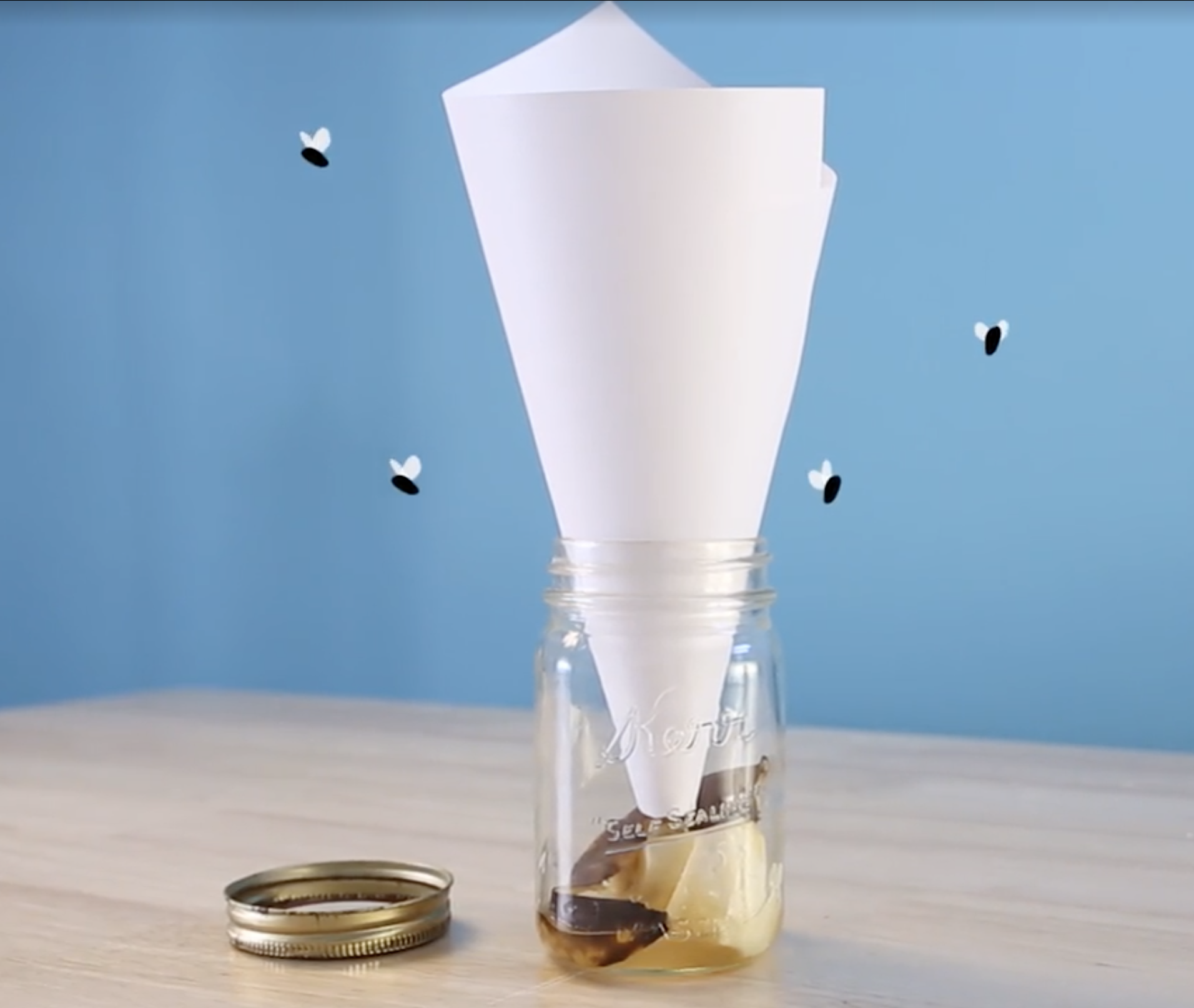This square-shaped color photograph features a homemade fly trap as its main subject. The scene is set against a medium blue background and a light blonde faux-wooden table surface characterized by horizontal striations. Central to the image is a clear glass Kerr mason jar, which prominently displays its brand name inscribed on the front. Inside the jar, at the bottom, lies a gold object, and possibly a paper towel soaked in a sugary substance. A piece of standard letter-sized paper, folded into a funnel shape, extends from the top of the jar, with its narrow end pointing inside, resembling a classic flytrap design. Beside the jar on the table sits its lid. Surrounding the jar are four small abstract representations of flies in white and black, enhancing the flytrap theme.